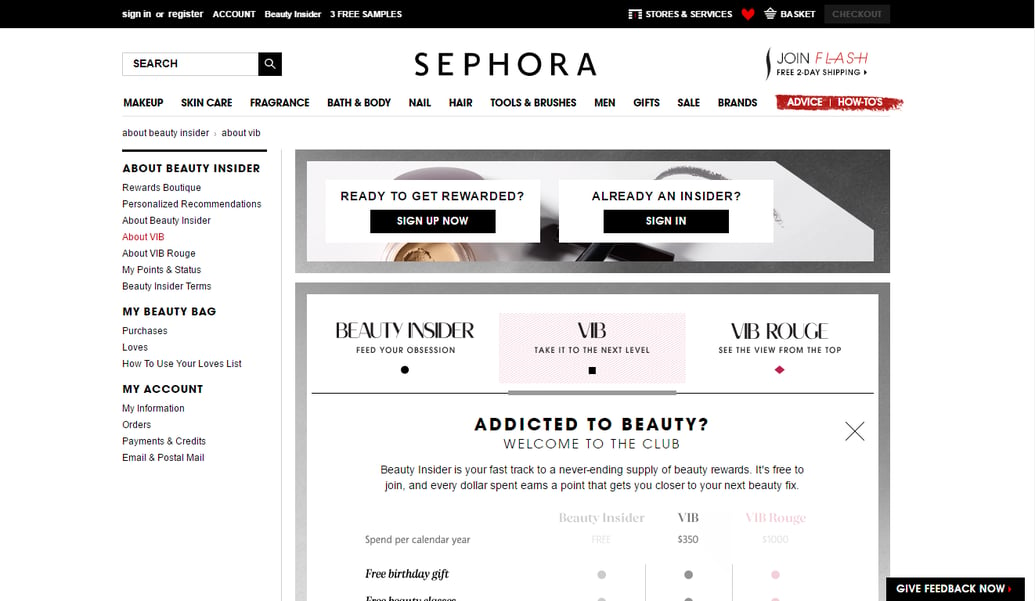Discover the ultimate beauty destination at Sephora, where you can explore an extensive range of makeup, skin care, fragrances, bath and body products, nail care, hair care, tools and brushes, and men's grooming essentials. Find products from all your favorite brands, and enjoy expert advice and tutorials on how to achieve your beauty goals. 

Join the Beauty Insider program to start earning rewards and receive exclusive perks. Whether you're a newbie or a VIB Rouge member, get ready to indulge in your beauty addiction. Sign up now to become a member, or sign in if you're already part of the club. With the Beauty Insider program, every dollar spent gets you closer to your next beauty fix, and you'll be able to track your progress and rewards on your personalized calendar. 

Don't miss out on free gifts, exclusive sales, and the chance to give feedback to shape the future of Sephora. Manage your account and keep your beauty bag updated to ensure you never run out of your favorite products. Join the Sephora community today and connect with fellow beauty enthusiasts on Facebook.